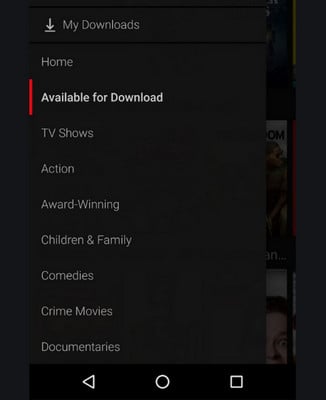The image shows a mobile interface with a black background, prominently displaying the "My Downloads" section in white text. There is an icon featuring a downward arrow with a line underneath it, signifying available downloads. To the left of this icon, a thin vertical red line adds a touch of color to the predominantly monochrome display.

At the top of the screen, a navigation option labeled "Home" allows users to return to the main page. The content suggests it might be from Netflix, as recognizable movie artwork for actors like Seth Rogen and Vince Vaughn is visible. Other movie artwork, resembling DVD covers, is displayed to the right.

Below the "Available for Download" section, various categories are listed, including TV Shows, Action, Award-Winning Movies, Children and Family, Comedies, Crime Movies, and Documentaries.

This screenshot is taken from a smartphone, evident by the navigation icons at the bottom: a triangle pointing left (Back button), a circle (Home button), and a square (Recent apps). The background beyond the "My Downloads" menu is slightly blurred, indicating an ongoing session with multiple options visible in a grayed-out form.

The user appears to be in the process of selecting a movie previously downloaded, highlighting the versatility and convenience of the streaming service, which could be Netflix, Hulu, or a similar platform.